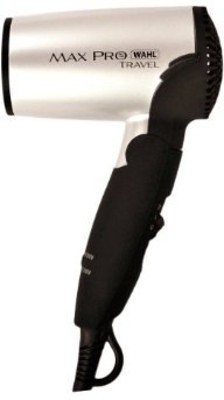The photograph features a compact handheld hairdryer prominently set against a pristine white background, emphasizing the device. The hairdryer, branded as "Max Pro Travel, W-A-H-L" in black letters along its side, showcases a sleek design. It has a small black handle that seamlessly blends into the black trims at both the back, where the fan motor is, and the very tip. The central body of the hairdryer, where the blower motor operates, is a shiny whitish-silver or chrome color, adding to its modern aesthetic. Visible on the left is a button or switch likely used for powering the device on and off or adjusting settings, which might include air intensity and heat levels. The power cord extends from the bottom but fades out of focus. The exclusive focus on the hairdryer against the plain backdrop accentuates its detailed design and compact form, making it the sole subject of the image.